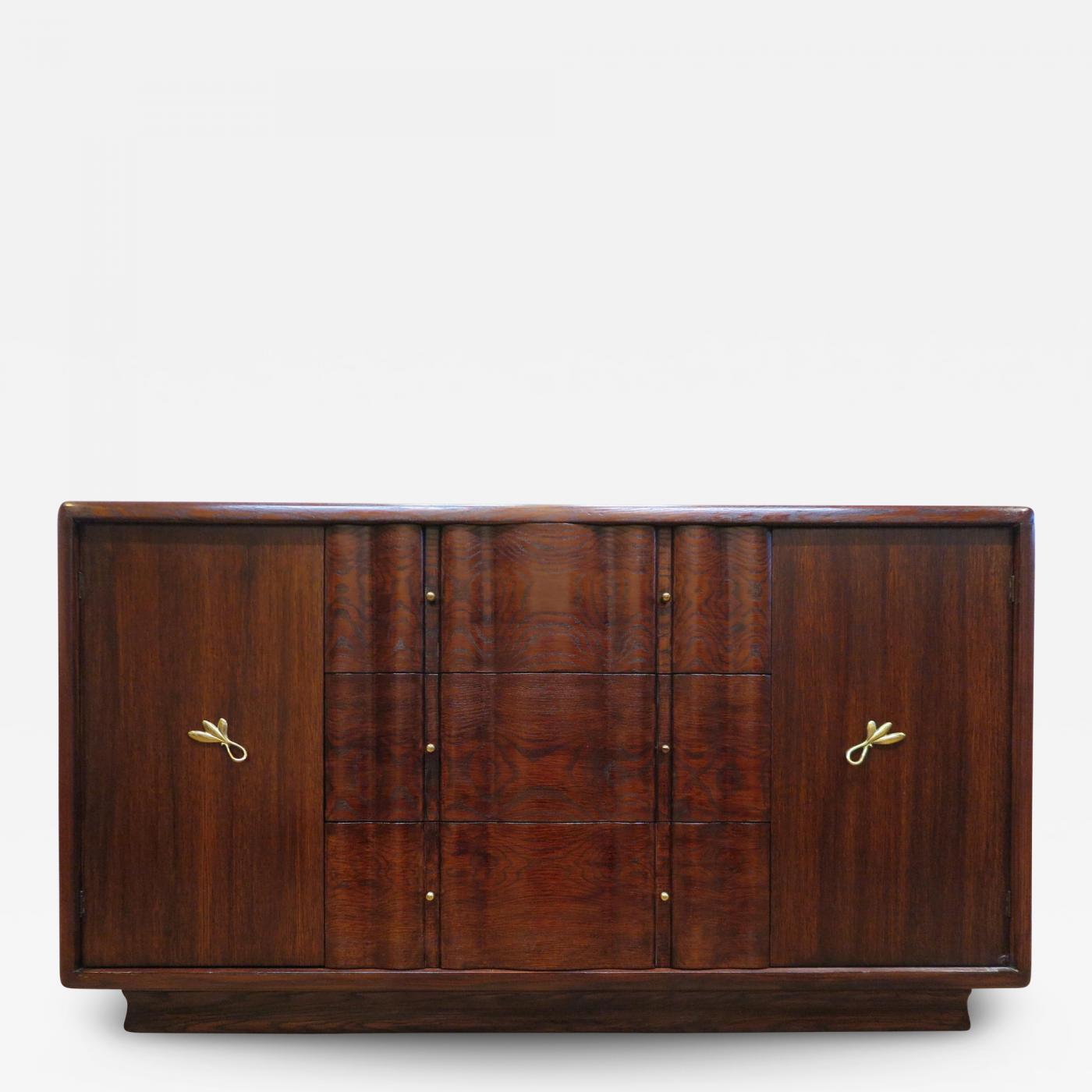The image depicts a highly detailed, dark mahogany chest of drawers, captured in a portrait-oriented color photograph with a style emphasizing realism and product photography. Central to the composition is the chest, featuring a reflective surface and a distinctive curved front. It consists of three horizontal drawers in the middle, each adorned with two small, round brass knobs. On either side of these drawers are vertical panels or doors, each equipped with ornate brass handles designed in a bow-and-leaf motif. The chest is elevated on a base that is slightly smaller than the top, adding to its elegant design. The background is a light gray or white, enhancing the chest’s rich wood grain and intricate details. The floor beneath the chest is also wooden, and there's a subtle shadow that adds depth to the overall image.